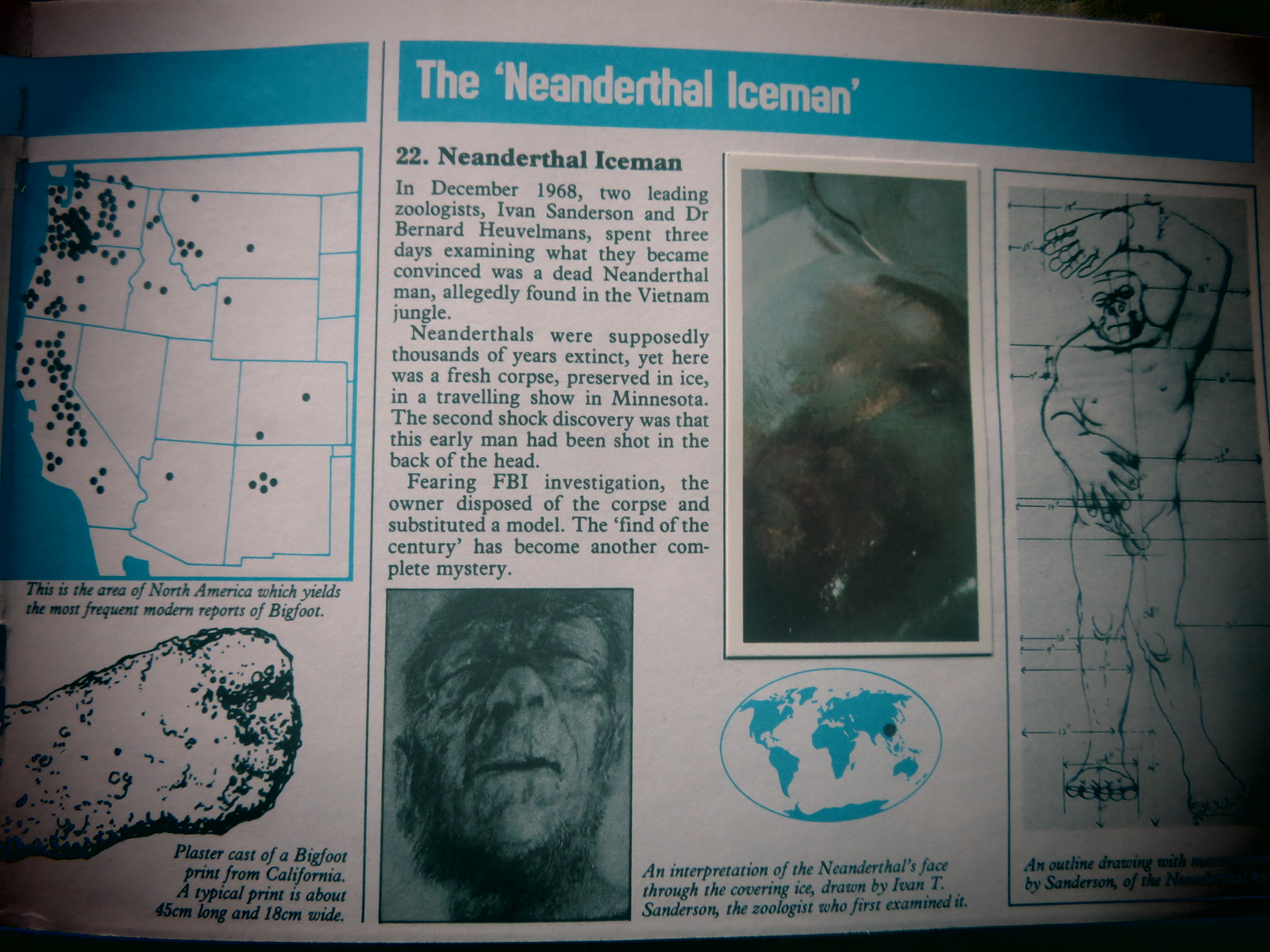The image depicts an informational placard titled "The Neanderthal Iceman" in white text against a blue banner at the top. The left side features a map of the United States with multiple dots, primarily in California and Washington. Below the map, there's a gray outline of a footprint, labeled as a plaster cast of a Bigfoot print from California, typically measuring about 45 centimeters long and 18 centimeters wide. 

Central to the placard is the number 22 alongside the heading "Neanderthal Iceman." The main article explains that in December 1968, zoologists Ivan Sanderson and Dr. Bernard Heuvelmans spent three days examining what they believed to be a dead Neanderthal man found in the Vietnam jungle. Despite Neanderthals being thought extinct for thousands of years, the fresh corpse preserved in ice was allegedly part of a traveling show in Minnesota. It was further revealed that this early man had been shot in the back of the head. To avoid FBI investigation, the corpse's owner replaced it with a model, turning what could have been the find of the century into an enduring mystery.

Below the column of text is an image of an old, wrinkled face, purportedly that of the Neanderthal Iceman. To the right of the face image, another blurry photograph is visible, and further down, there's a hand-drawn diagram of a naked Neanderthal Iceman. Additional writings spread throughout the placard offer more context, with captions indicating frequent modern reports of Bigfoot in North America.